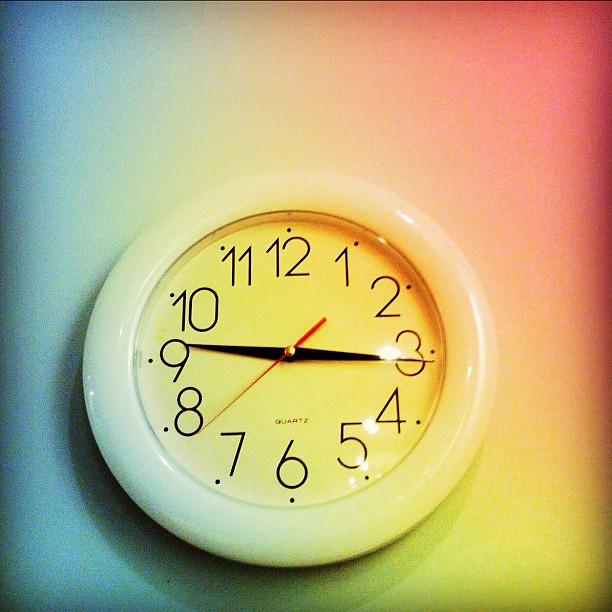A close-up image of a wall-mounted clock prominently features the clock face slightly off-center, positioned towards the lower left of the frame. The wall behind the clock is bathed in a gradient filter, transitioning from deep blue on the left to a lighter blue, then to a greenish-yellow hue. On the right side of the image, the background transitions from green at the bottom to a peach, and then to a pinkish-red at the top. The clock, encased in a white plastic frame, has a face with a subtle yellow hue. The black hour and minute hands indicate the time is quarter to three, while a red second hand points to the eight. Surrounding the outer border of the clock face are black hour numbers, each accented with a small black dot.